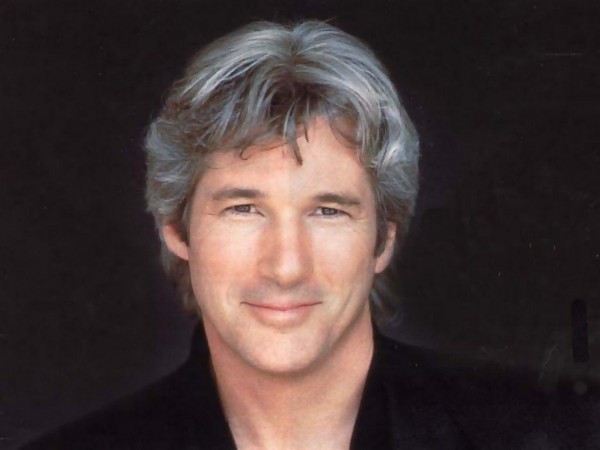This is a close-up, grainy photograph of the actor Richard Gere, known for his roles in "An Officer and a Gentleman" and "American Gigolo." The image captures him from the shoulders up, standing against a solid black backdrop, drawing all attention to his face. Gere is dressed in a black top, which could be a suit jacket or robe with nothing worn underneath, giving a minimalist yet striking appearance. He has his head slightly bent, looking directly at the camera with a slight, closed-lip smile. His hair, a characteristic salt-and-pepper mix, is medium-length and parted down the middle, with some strands gently hanging over his ears. His brown eyes and matching eyebrows add to his familiar, distinguished look. The overall impression is of a timeless, introspective moment frozen in a photograph that blends both past and present elements of Gere's enduring screen presence.